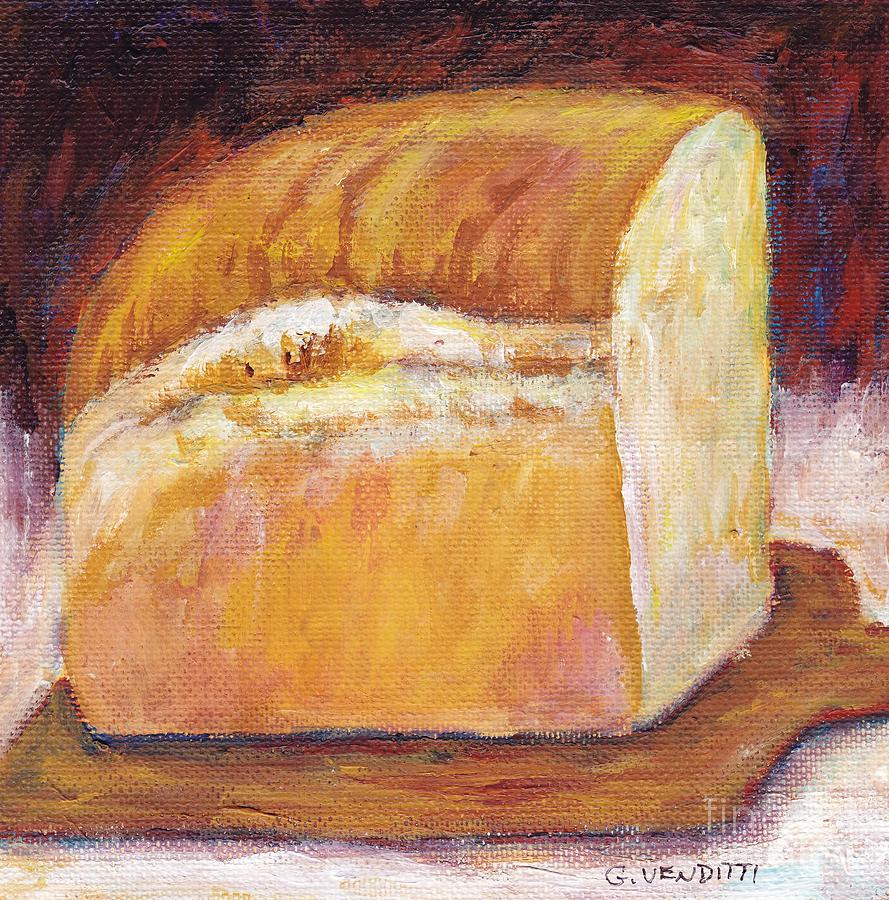This vertical rectangular painting depicts a rustic half loaf of bread seated on a small, square-shaped wooden cutting board, which appears to be a paddle used for baking. The loaf, characterized by its squat and tall shape, showcases a golden-brown crust with crusty details created using splashes of orange and brown paint. The interior of the loaf is white and mottled, suggesting a home-baked quality. The surrounding surface is a whitish-orange color, adding to the rustic ambiance of the piece. The background above the loaf features dark reddish-blue strokes, consistent with an Impressionistic style marked by fast, broad strokes. Notably, the lower right corner of the painting is signed "G. Venditti" in black paint, further emphasizing the artwork's country feel.